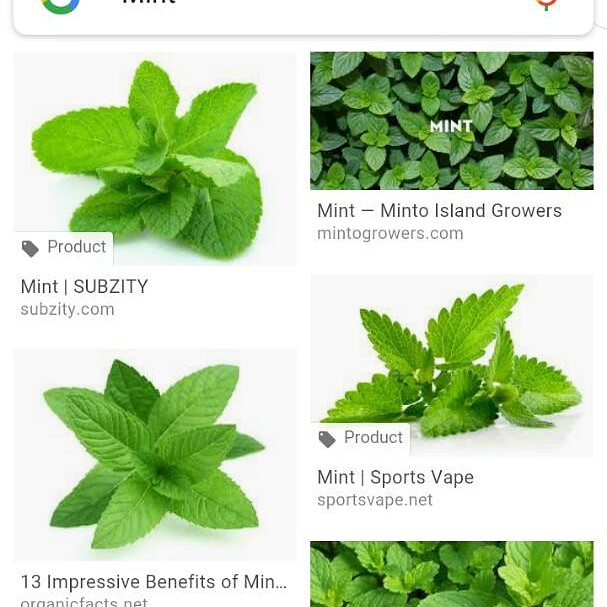This image depicts a screenshot of a Google image search focused on mint. The screen displays five distinct pictures of mint leaves arranged in two columns, with two images on the left and three on the right. Each image portrays mint in various perspectives, some zoomed in to highlight the sprigs. Underneath each image, there are snippets of text providing the titles and sources of related articles or websites. The titles include "Mint Subsidy" from subsidy.com, "Minto Island Growers" from mintogrowers.com, "13 Impressive Benefits of Mint" from organicfacts.net, and "Mint Sports Vape" from sportsvape.net. One of the images has its text cut off, leaving only the mint leaves visible. These snippets suggest clickable links that would direct users to specific articles or products related to mint.